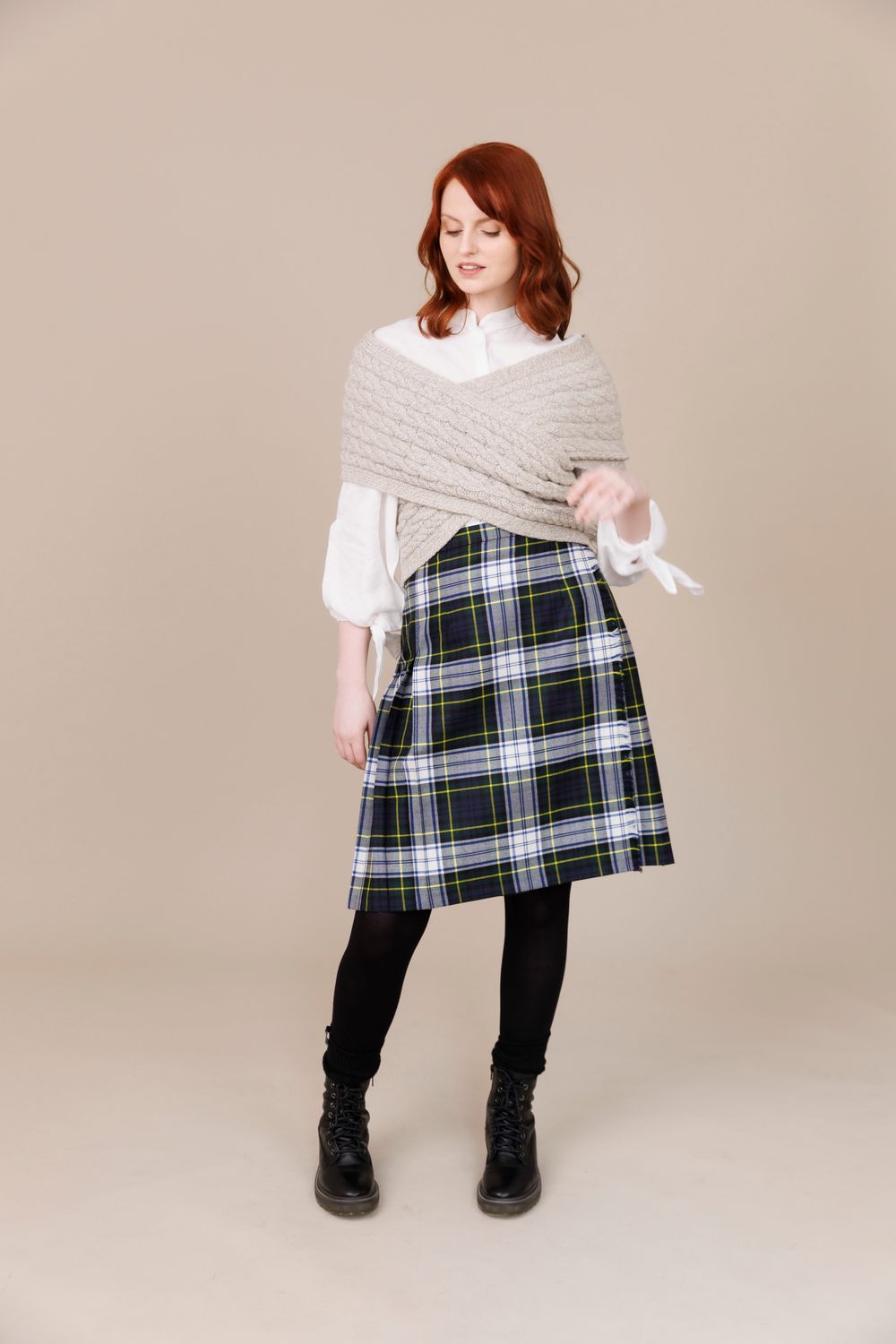The image captures a striking fashion photograph featuring a female model who has vibrant auburn hair cascading in soft waves to her shoulders, accentuated by a side bang. She stands in the center of what appears to be a meticulously staged photographic setup, characterized by smooth, pale beige walls and floor that seamlessly blend together, thereby directing all attention to her. The model exudes a vintage charm, reminiscent of Scottish aesthetics, with her attire consisting of a white blouse with puffy sleeves and a beige, wrap-around knitted shawl draped over her shoulders. Her outfit is completed by a pleated, tartan skirt in shades of green, white, and touches of yellow, paired with black over-the-knee boots that emphasize her poised stance. Her black leggings peek from underneath the skirt, adding a modern twist to the classic ensemble. The model's head is tilted slightly downwards with a subtle, serene smile gracing her lips, and her left hand displays a blur, suggesting a moment captured in motion. Her delicately painted reddish-pink fingernails add a final touch of elegance to the image.